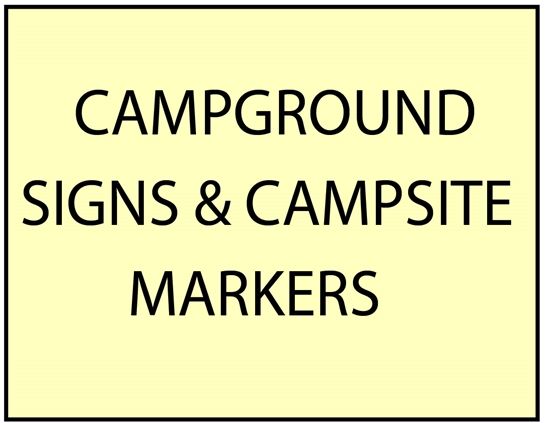The image features a plain, light yellow background with a thin black border framing it. Centered on the image, there is bold, uppercase black text that reads "CAMPGROUND SIGNS AND CAMPSITE MARKERS." The text is the focal point, arranged neatly one line on top of the other, giving the appearance of a sign or a posted notice. There are no other objects or visual elements in the image, enhancing the text's visibility and impact. The combination of yellow, black, and white creates a strong contrast that makes the message stand out clearly. This could be a sign you'd find at a campground, in a store, or on a website related to camping.